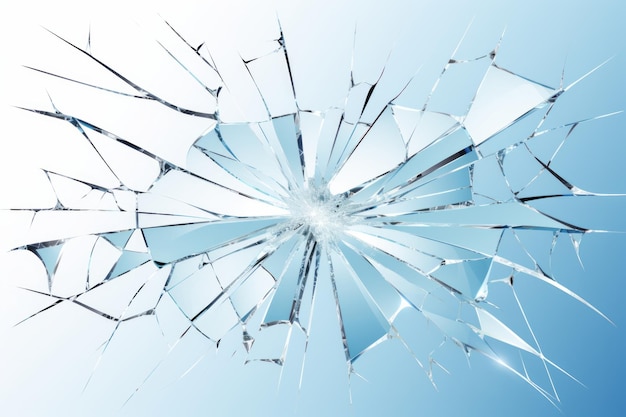The image depicts a horizontally oriented, standard 4 by 3 ratio piece of glass that has been shattered, with the center of the impact located precisely in the middle of the frame. From this central point, numerous cracks radiate outward, creating a web-like pattern. The glass, which is predominantly blue, transitions from a bright, almost white hue in the top left corner to a much darker, deep blue in the bottom right. This gradient suggests a light source positioned on the left side of the image, casting a progressively darker shadow towards the right. The shattered glass forms intricate shapes, including upside-down triangles, sideways triangles, rectangles, and pentagons, particularly noticeable towards the edges. The detailed cracks and shards converge in a dense, chaotic pattern at the center, while some of the cracks form thin, bright white lines that extend towards the edges, eventually thinning out. The appearance of some geometric shapes and patterns suggests a potential combination of both real and computer-generated elements, enhancing the complexity of the shattered glass depiction.